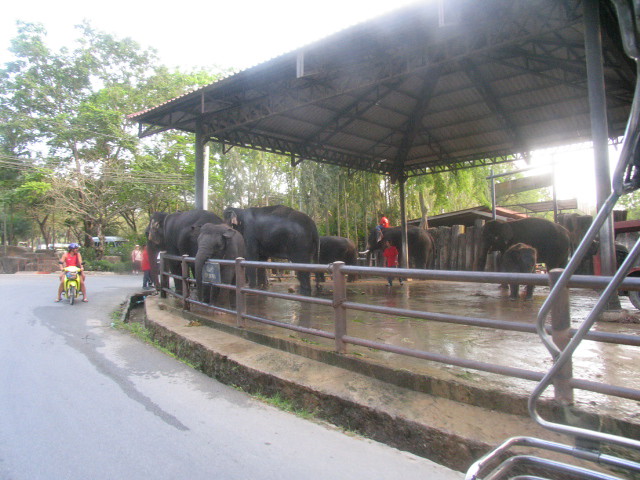The photograph captures a vivid scene at what appears to be an outdoor zoo or elephant sanctuary. Central to the image is a large, rectangular enclosure, roughly 30 feet by 30 feet, with a concrete floor and metal bars surrounding it. A substantial metal canopy provides shade to the enclosure. Inside, there are notably seven elephants, comprising both adults and calves of varying ages. The sun streams in from the back, casting a bright light over the scene.

A person in a red shirt and blue jeans is seen among the elephants, possibly a caretaker. Some elephants are seen leaning over the railings, suggesting interaction with onlookers. Outside the enclosure, the area is surrounded by vibrant green trees and grass. A road or pathway winds around the enclosure, where a person in a red shirt rides a yellow scooter, pausing to look at the elephants. The photograph is oriented horizontally and seems to have been taken on a clear, sunny day, evidenced by the bright white sky and visible sunlight.